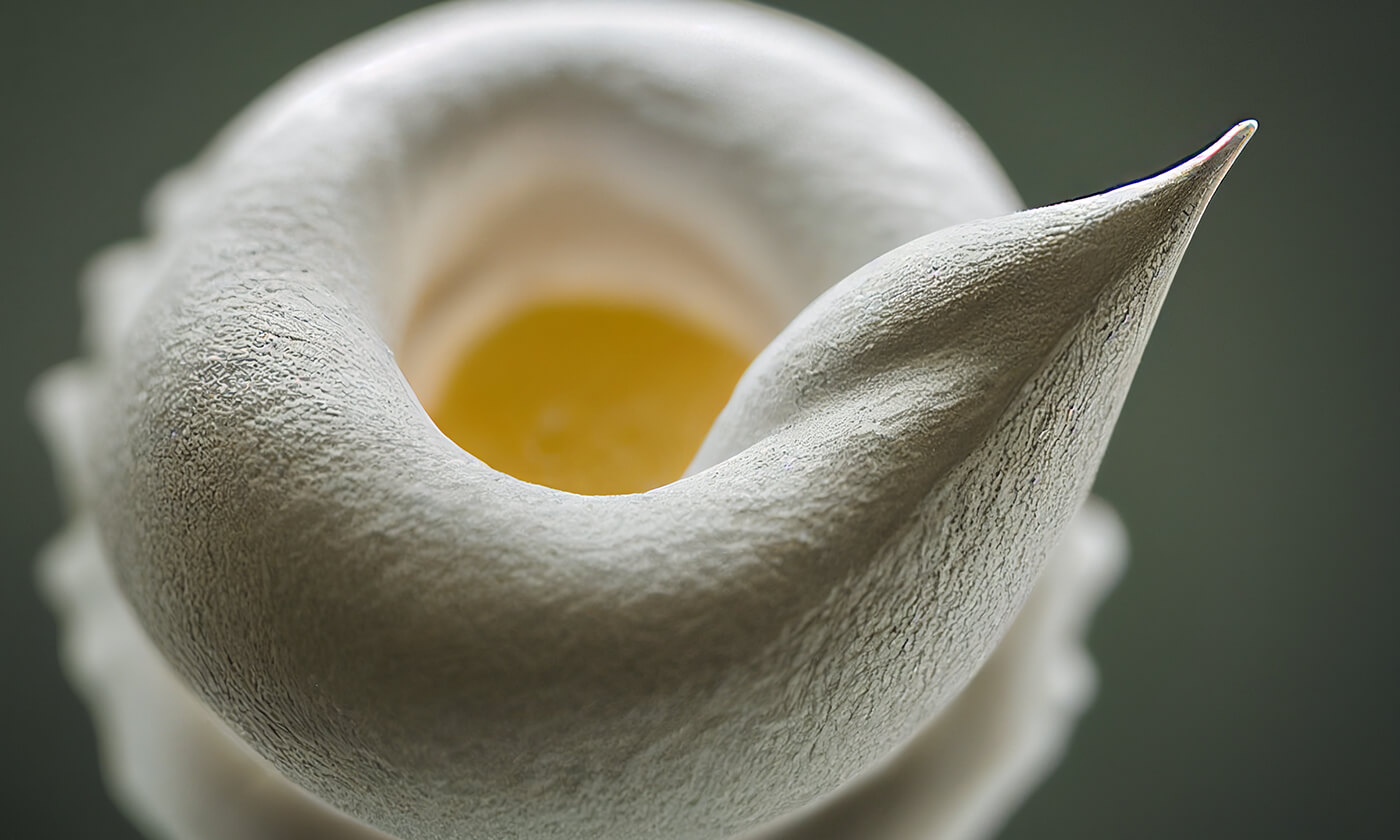The image appears to depict a meticulously crafted culinary creation resembling stiffly beaten egg whites, sculpted into a tall, circular formation with a hollow center, akin to a donut shape. The structure's base seems to have been spun from top to bottom, lending it height and a graceful taper. Remarkably, the upper part of this creation culminates in the delicate form of a bird's side profile, complete with a beak. Inside this tunnel-like structure, nestled at the bottom, are rich, golden-yellow egg yolks. The predominantly white object is accented with subtle light brown hues, adding depth and visual interest to the overall presentation.